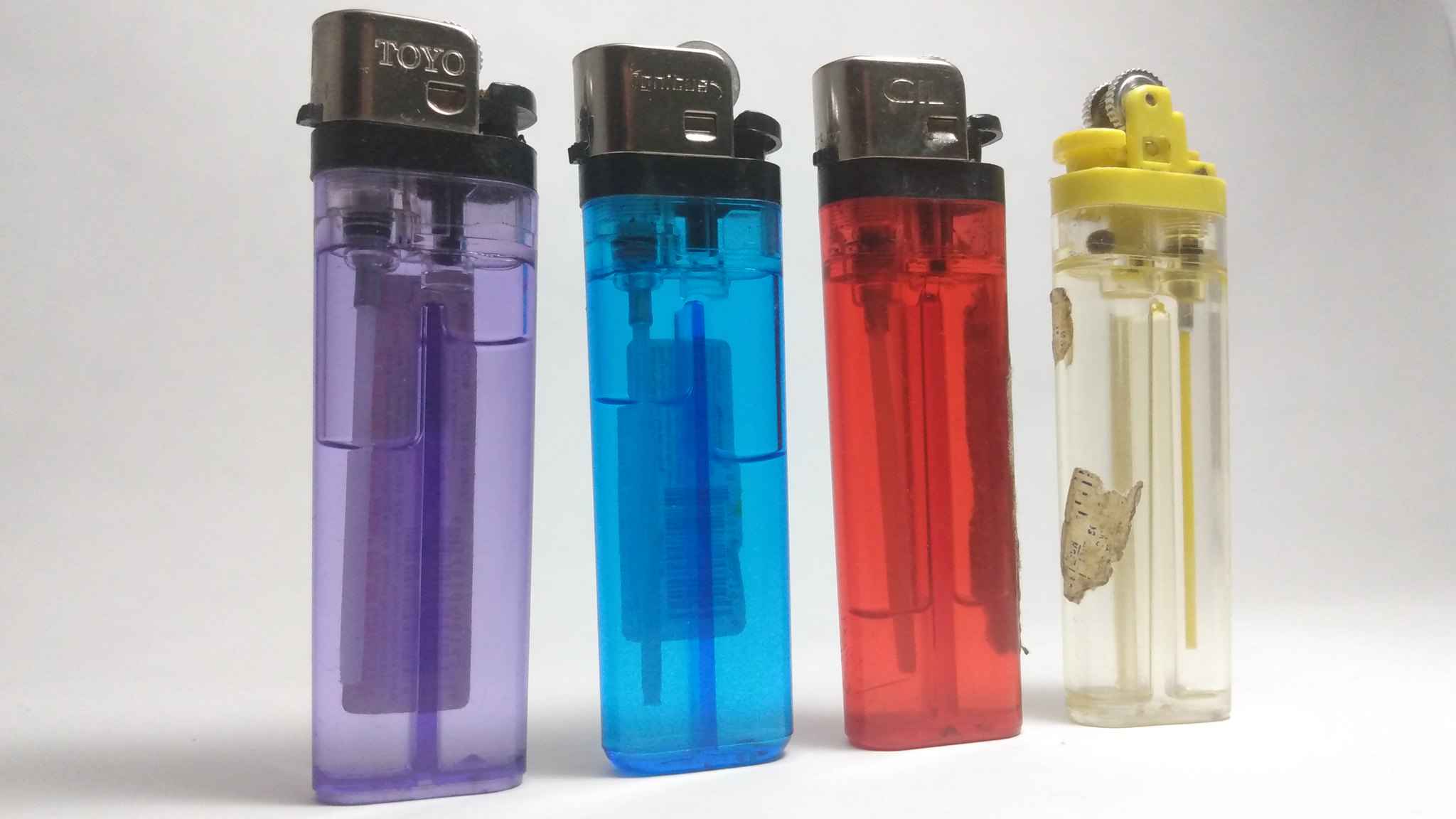This photograph showcases four transparent, disposable cigarette lighters standing upright in a row on a gray background. The lighters are arranged from left to right in the following colors: clear purple, clear blue, clear red, and clear with a yellow top. Each lighter, except for the fourth one, features a black rim at the top and a silver flame shield. The purple lighter has a "Toyo" brand logo visible, while the clear lighter with the yellow top has a silver igniter and a yellow straw inside for fuel intake. The detailed transparency of the lighters reveals their internal mechanisms. A shadow is cast at the bottom, adding depth to the centered composition.